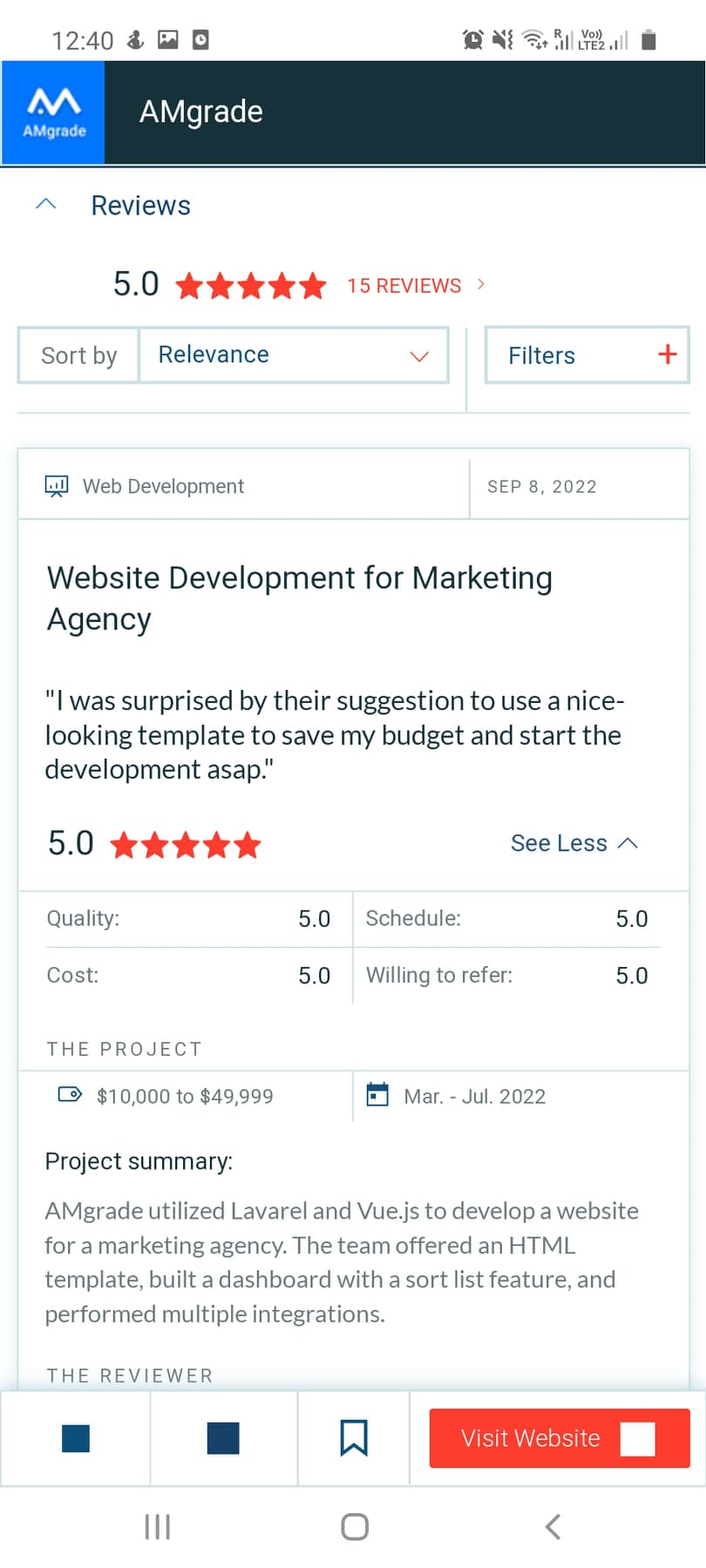**Screenshot Caption: Detailed Interface Overview**

This screenshot captures a tablet or smartphone screen displaying various interface elements in military time (12:40). The status bar at the top shows numerous icons: a running person silhouette, a screenshot icon, a watch-like icon, and a clock indicating an alarm is set. Additionally, there's a speaker icon with a line through it (silenced), strong WiFi signal, roaming cell phone signal, LTE2 with 2 out of 4 bars, and an almost full battery symbol.

In the middle of the screen, within a dark blue rectangle, there's a segment featuring a slightly lighter navy blue square with a bold white 'M' (resembling mountains) and a small white dot on the left. Below this, it says "A-M-G-R-A-D-E" in white, indicating AMS grade, with "AM grade" repeated on the right side in darker blue.

Beneath this, a cyan arrow pointing upwards accompanies the word "reviews" in blue. Below, the text "5.0" in black is followed by five red stars, "15 reviews" in red, and a right-pointing red arrow. 

A light blue/dark gray rectangle shows "sort by" in dark gray on one side, and "relevance" in bold blue with a red drop-down arrow on the other. Adjacent to it, another rectangle in dark blue says "filters," and a red plus sign is on the right.

A larger bordered rectangle features a blue monitor/presentation icon, with "web development" in thin gray text next to it. To the right, "SCP-8-2022" signifies September 8th, 2022. Below, in bold black text, it says "website development for a marketing agency," followed by a quoted testimonial: "I was surprised by their suggestion to use a nice looking template to save my budget and start the development ASAP." This review is rated 5.0 stars, complete with five red stars.

On the right, bold thin blue text "see less" with an up arrow directs the user to collapse the section. Additional ratings under this include quality (5.0), schedule (5.0), cost (5.0), and willingness to refer (5.0). 

The product section, marked by a blue tag icon, mentions a price range of 10,000 to 49,999. To the right, a blue calendar icon with "MAR-JUL 2022" in gray highlights the project duration.

The bold black "product summary" title is followed by details stating that AM grade utilized LAVAREEL and VUE.js for the project, built an HTML template, dashboard with list features, and performed multiple integrations.

At the bottom, the reviewer section features a bezel with two dark blue squares and a bookmark symbol. Lastly, an orange rectangle with white text "visit website" alongside a white square invites further action.